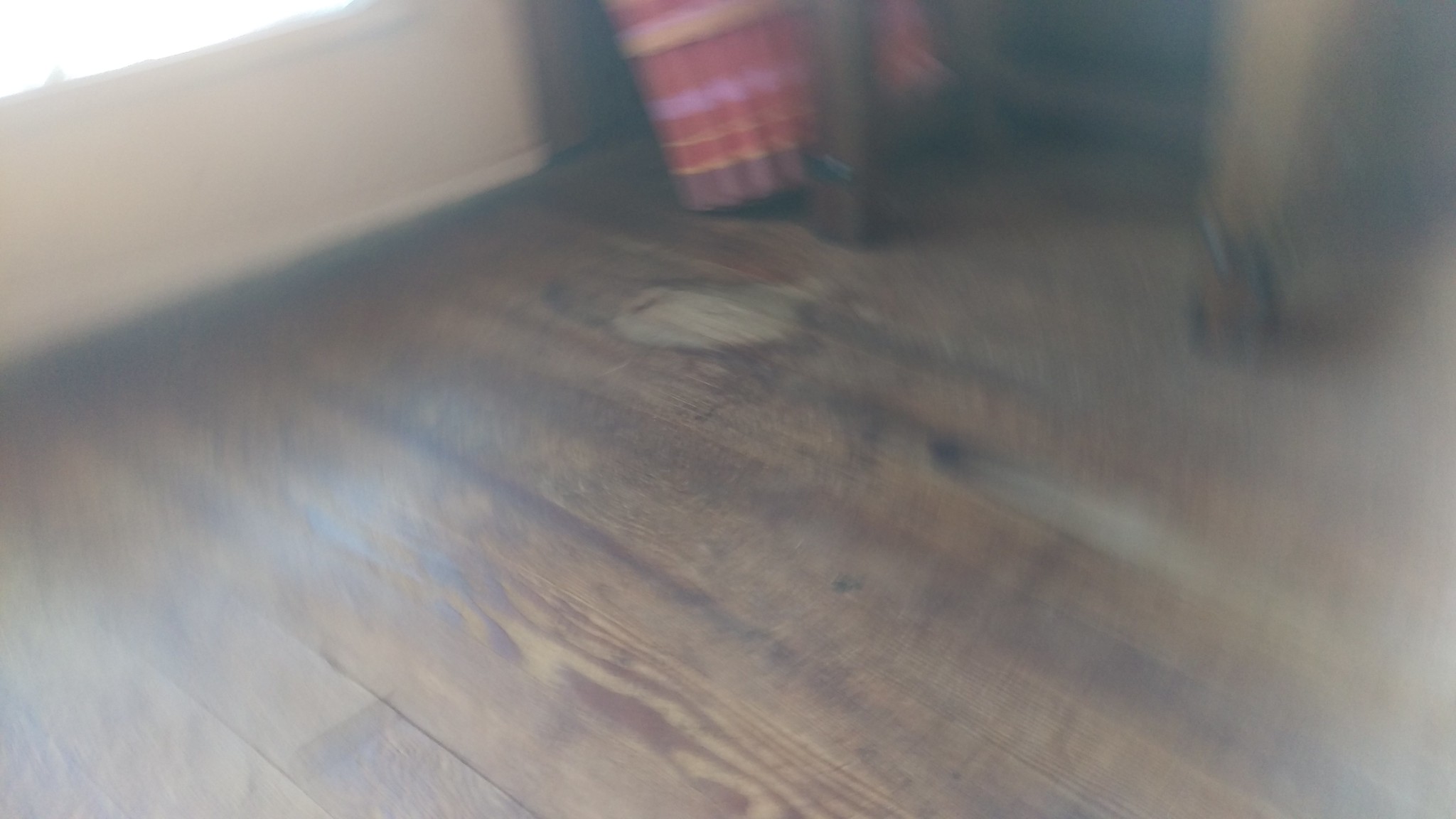This is a blurry photograph of a rustic dark wood floor with noticeable radial smudging, suggesting the camera was twisted as the picture was taken. The floor, which has prominent knots similar to those found in trees and a conspicuous stain possibly caused by water damage, is the main feature of the image. The edges of the picture are significantly more blurred than the center. Towards the top left, there's a white door or wall, illuminated by some brighter light that might be coming from a window. In the top right, there appears to be a cluster of brown objects which seem to be chair legs, one notably lighter than the others. Additionally, there is a rolled-up blanket leaning against the wall, and a red and brown object which may be part of a curtain.